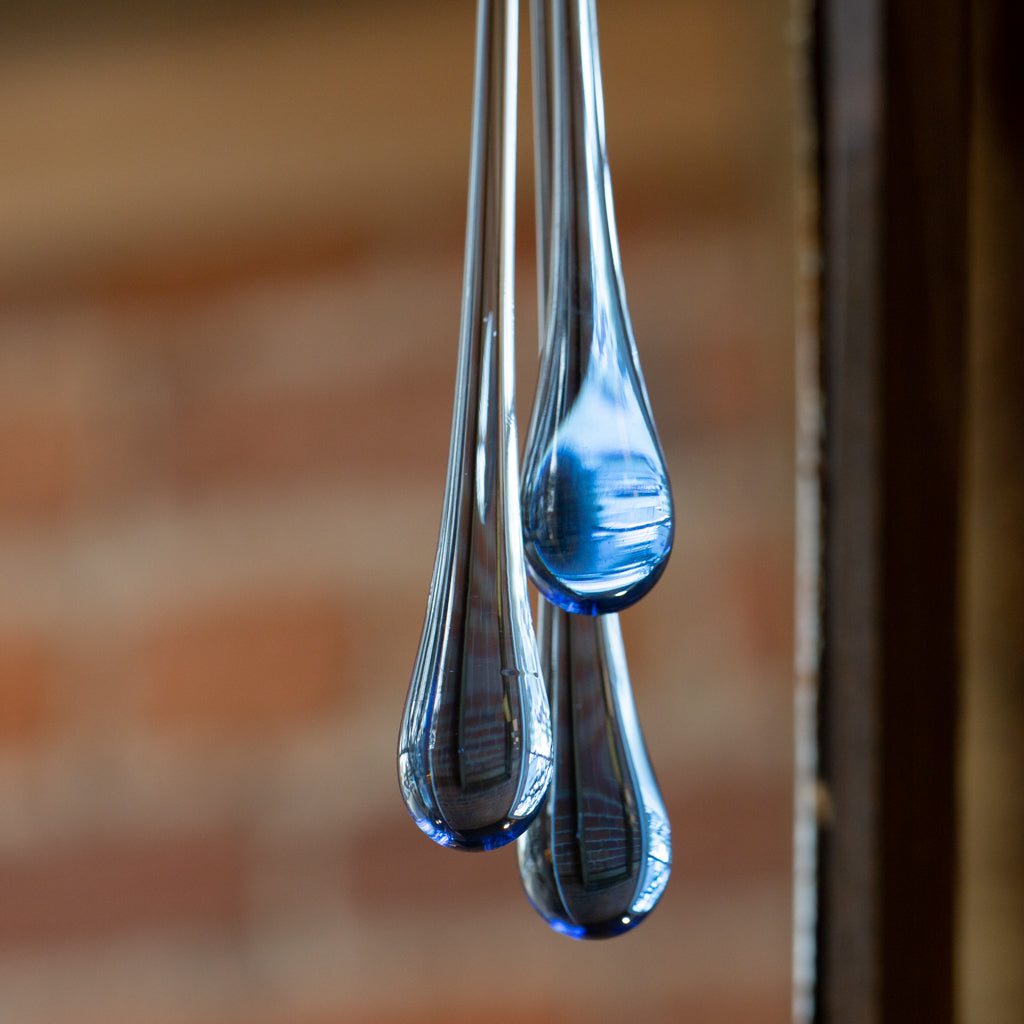In this close-up image, three elongated droplets hang suspended against a blurred, brownish background, showcasing a mesmerizing play of light and reflections. The foremost droplet, which hangs the highest, is distinctly blue, capturing and reflecting a light source that gives it a vivid tint. The second droplet, positioned between the foreground and background, and the third, which hangs the lowest, both carry a more subdued, grayish-brown hue with white reflections. The droplets taper as they extend upwards, bulging at the bottom in a manner characteristic of liquid drops, though their elongated form suggests they may not be water. Within the reflections of the middle and back droplets, a brick wall and a golden frame-like object are visible, suggesting an intriguing setting. To the right of the droplets, there's a hint of a metal bar, possibly part of a faucet, though the focus remains primarily on the captivating droplets themselves.